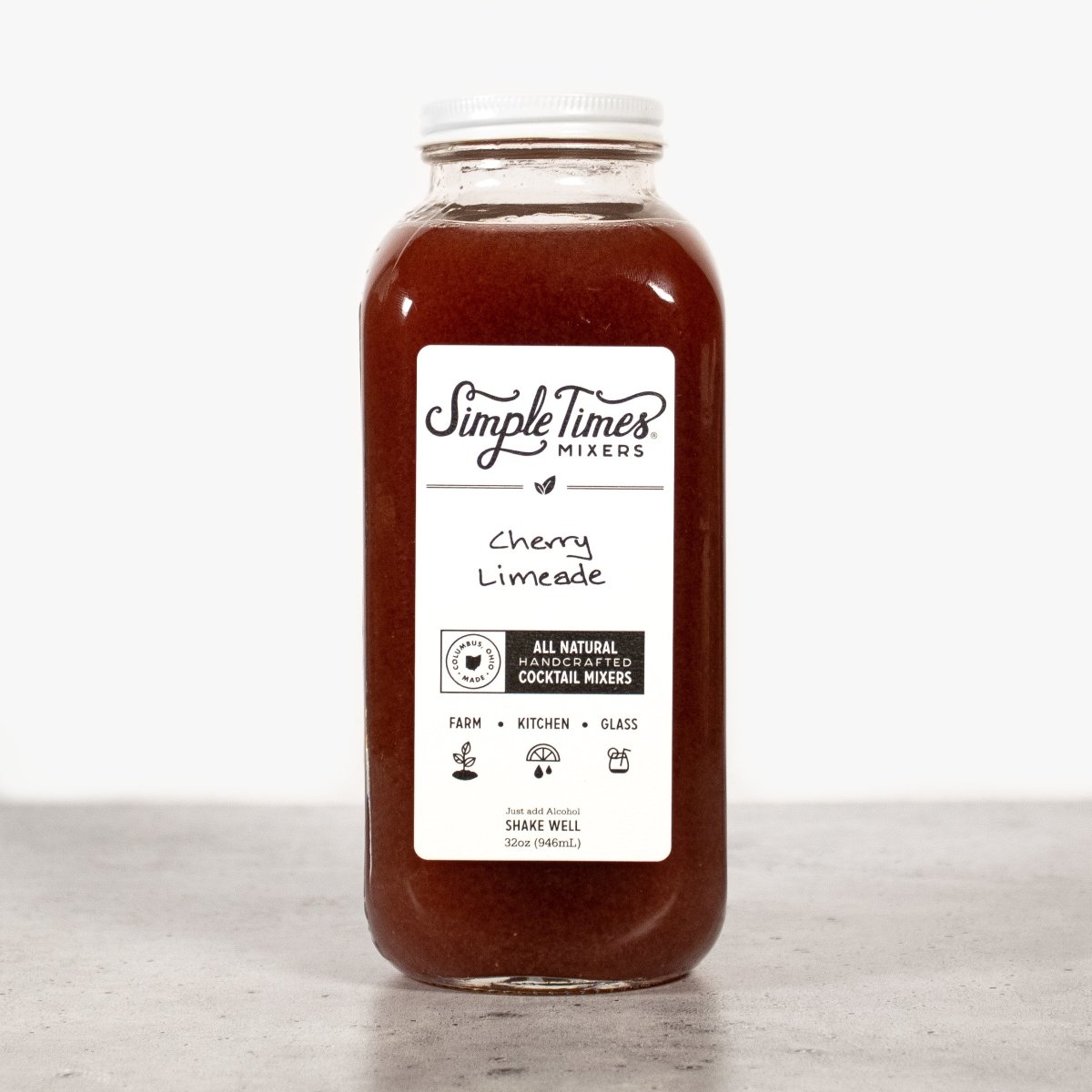This image features a clear, square mason jar with rounded corners filled with a deep red liquid, identified as a handcrafted, all-natural cocktail mixer by the label. The jar is sealed with a white screw cap and prominently displays a white label. The label reads "Simple Times Mixers" at the top, followed by "Cherry Limeade." Underneath, it states "All Natural Handcrafted Cocktail Mixers." The label also features icons representing "Farm," "Kitchen," and "Glass," along with instructions to "Shake Well." The jar is set against a backdrop of a white wall and a gray surface, suggesting it rests on a table. This vertical image captures the jar in the center, offering a clear view of the vibrant maroon liquid inside.